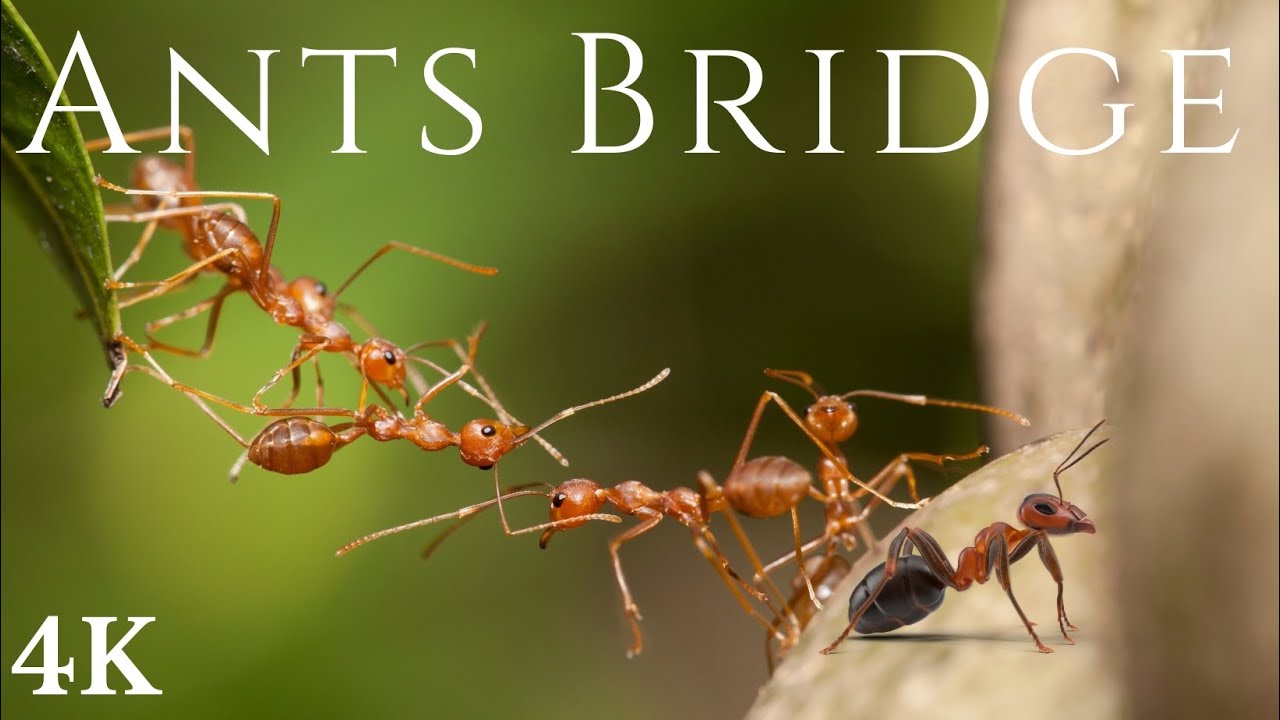In this high-resolution 4K color photograph, a close-up view captures a group of red ants forming a living bridge. The image features the words "Ants Bridge" in large white text at the top. In the upper left corner, the tip of a green leaf can be seen. A single ant clings to the leaf, holding onto another ant with its mandibles. This chain of ants dangles in the air, stretching towards a light beige surface on the right, which appears to be some sort of rock. There are additional ants on this surface, contributing to the bridge. The background is a soft, out-of-focus green. The detailed visualization illustrates the remarkable cooperation among ants as they create a bridge to traverse a gap, highlighting their social behavior and collective problem-solving abilities.